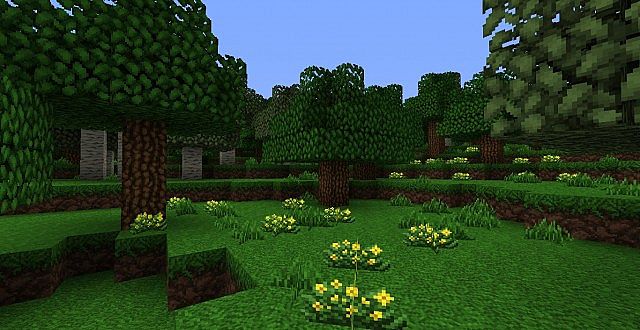The image appears to be a computer-generated depiction of a verdant landscape. The scene showcases a tiered green area, with each level descending to another lush green zone. The steps connecting the levels are adorned with patches of brown and green. The uppermost green area is dotted with blooming daffodils interspersed with patches of longer green grass. The tree trunks, rendered in dark brown with lighter brown patches, exhibit a uniform appearance, indicative of computer generation. The leaves are consistent across all trees, giving a sense of uniformity. The trees, angled to the left, appear to sway as if being blown by the wind. The arrangement continues as far as the eye can see, creating a repeating pattern of trees at different elevations, surrounded by alternating patches of grass and daffodils. The boxy nature of the tree trunks further emphasizes the artificial creation of the image.